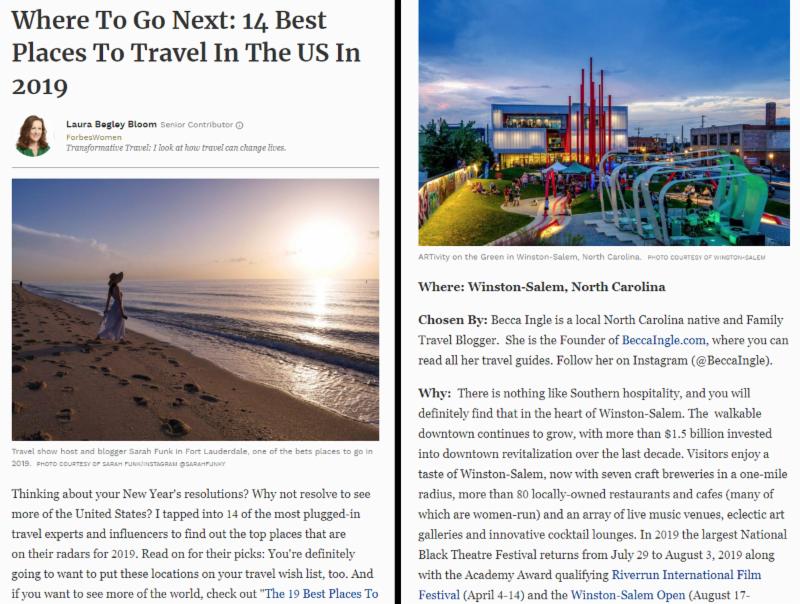**Descriptive Caption:**
In this captivating spread from Forbes Women, senior contributor Laura Bagley-Bloom introduces the "14 Best Places to Travel in the US in 2019." With her signature auburn curls, pale complexion, and chic green blouse, Laura, who is an advocate for transformative travel, shares her insightful recommendations.

The left side of the spread features a serene image of a lone woman in a hat, dressed in white, standing on a beach at sunrise. The tranquil scene exudes a sense of relaxation and freedom.

Highlighted as the first travel destination, Winston-Salem, North Carolina, shines through the lens of Becca Engel, a North Carolina native and family travel blogger. The accompanying image depicts Artivity on the Green, a modern art museum in Winston-Salem that doubles as an interactive playground.

Becca unveils Winston-Salem's charm, emphasizing its walkable downtown, seven craft breweries, and an impressive selection of 80 locally-owned, women-run restaurants and cafes. She paints a vibrant picture of the city's cultural scene, highlighting an array of live music venues, collective art galleries, and innovative cocktail lounges.

Furthermore, Becca mentions prominent events such as the National Black Theater Festival, occurring from July 29th to August 3rd, 2019, the Academy Award-qualifying RiverRun International Film Festival, and the Winston-Salem Open, making the city a must-visit destination.